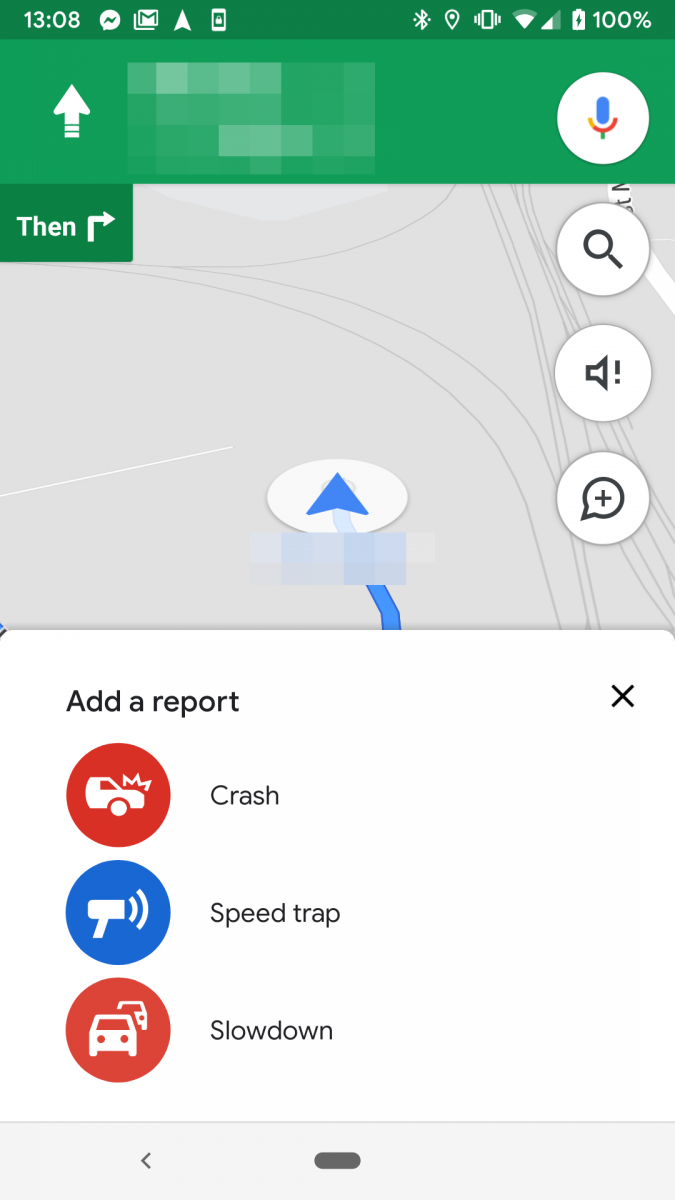The image depicts a smartphone interface with various icons and notifications. The screen shows multiple app icons, including Facebook, Messenger, and Gmail. Along the top of the display, there are several status indicators: a Bluetooth symbol, location symbol, vibrate mode icon, Wi-Fi signal with two out of four bars, and a full 100% battery indicator.

On the screen, there's an upload arrow, a microphone icon, a right-turning arrow, a search icon, and a speaker with an exclamation mark. Additionally, there is a circular icon with a plus sign in the center and another white circle containing a blue arrow with a blue line trailing behind it. The lower portion of the screen is white, displaying the text "Add a report."

Further details include an 'Exit' option in the corner labeled "Crash", "Speed Trap", and "Slow Down." The "Crash" option is represented by an icon of a car hood with an explosion, "Speed Trap" by a bullhorn, and "Slow Down" by two cars, one tailing the other. At the bottom of the interface, there are 'Back' and 'Home' buttons.